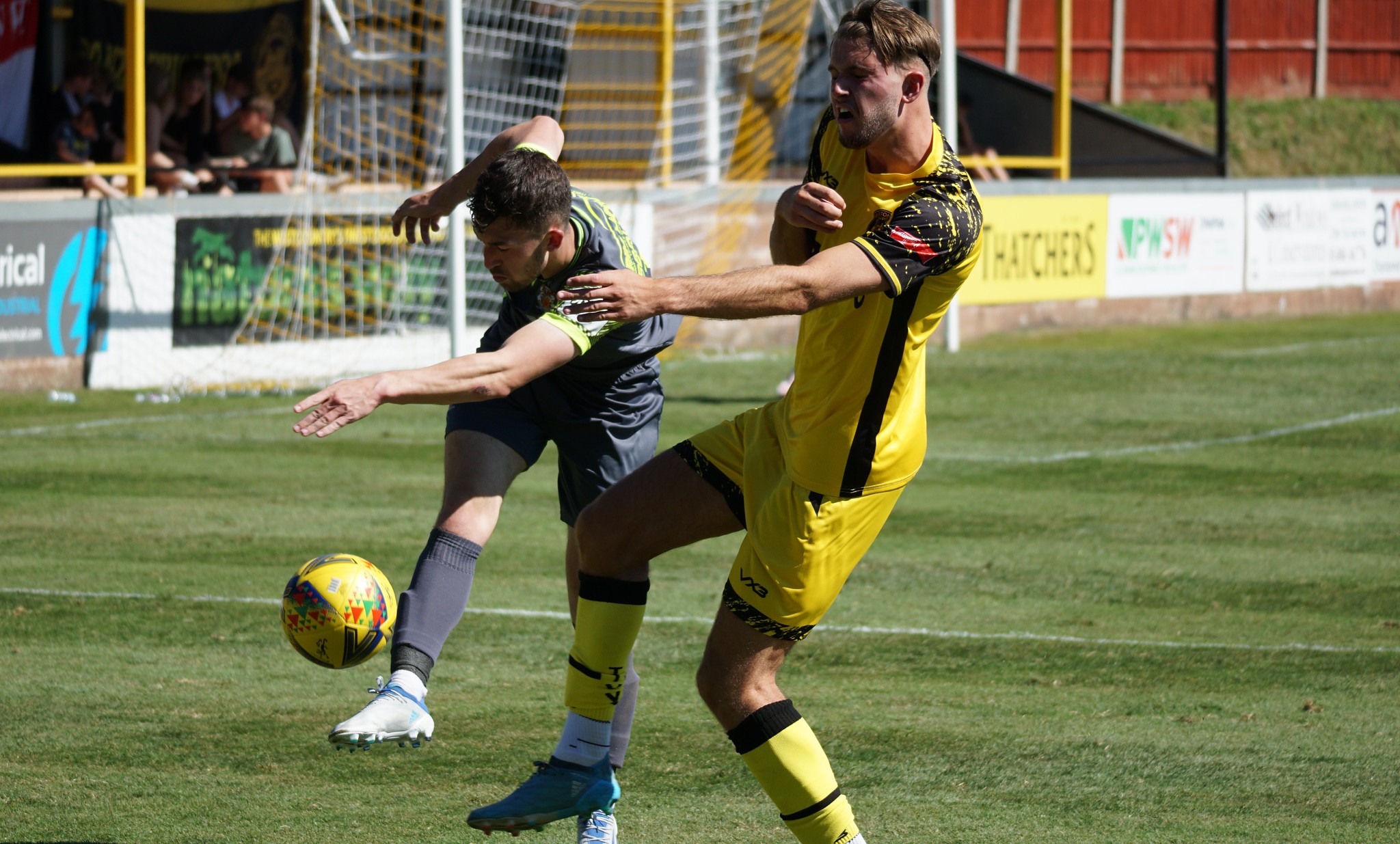In this vivid daytime scene on a green soccer pitch, two players are captured in the heat of play. The player in the foreground, centered in the image, is seen kicking a yellow soccer ball that's mid-air. He is fully decked in a striking yellow uniform with a yellow top featuring black sleeves and a black stripe, yellow shorts, yellow socks, yellow shin guards, and black soccer shoes. To his right, the other player appears in a somewhat awkward stride, possibly lunging to intercept the ball. This player is clad in a grayish-blue uniform complete with lime green lettering and accents, gray shorts, gray socks, gray shin guards, and white shoes. In the background, the goal with its white and yellow netting stands prominently, though without a goalkeeper. A few scattered spectators and signs, including one that says "Thatchers," line the distant edge of the pitch. The bright daylight suggests a sunny atmosphere, casting shadows on the field.